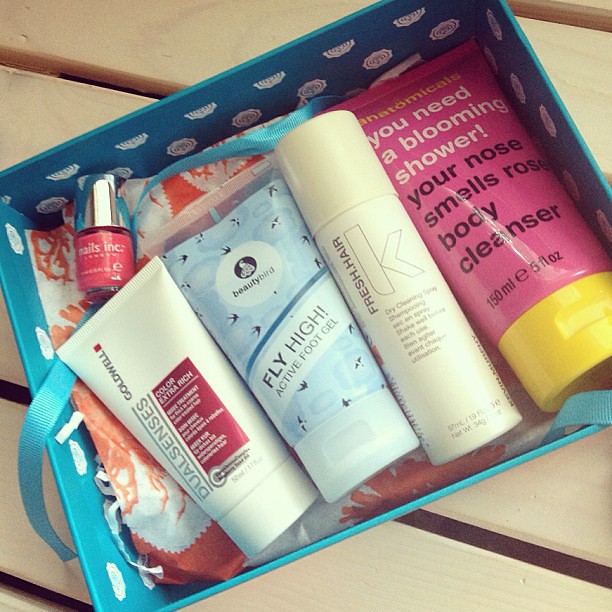This is a detailed photograph of a gift box containing an assortment of travel-sized toiletries, positioned on a wooden bench with diagonal slats. The light turquoise box, accentuated with a matching ribbon, holds items nestled in crumpled white and peach tissue paper. From left to right inside the box: a white tube labeled "Dual Senses Color Extra Rich," a light blue tube of "Beauty Bird Fly High Active Foot Gel" adorned with bird graphics, a light tan cylinder of "Fresh Hair K" dry shampoo, and a prominent pink tube with a yellow cap of "Anatomicals - You Need a Blooming Shower, Your Nose Smells Rosy" body cleanser. Additionally, a bottle of Pink Fianna Polish with a silver cap is situated above the Dual Senses cream. The gift box's interior also features a possible crown motif with white circular elements, adding a touch of elegance to the presentation.